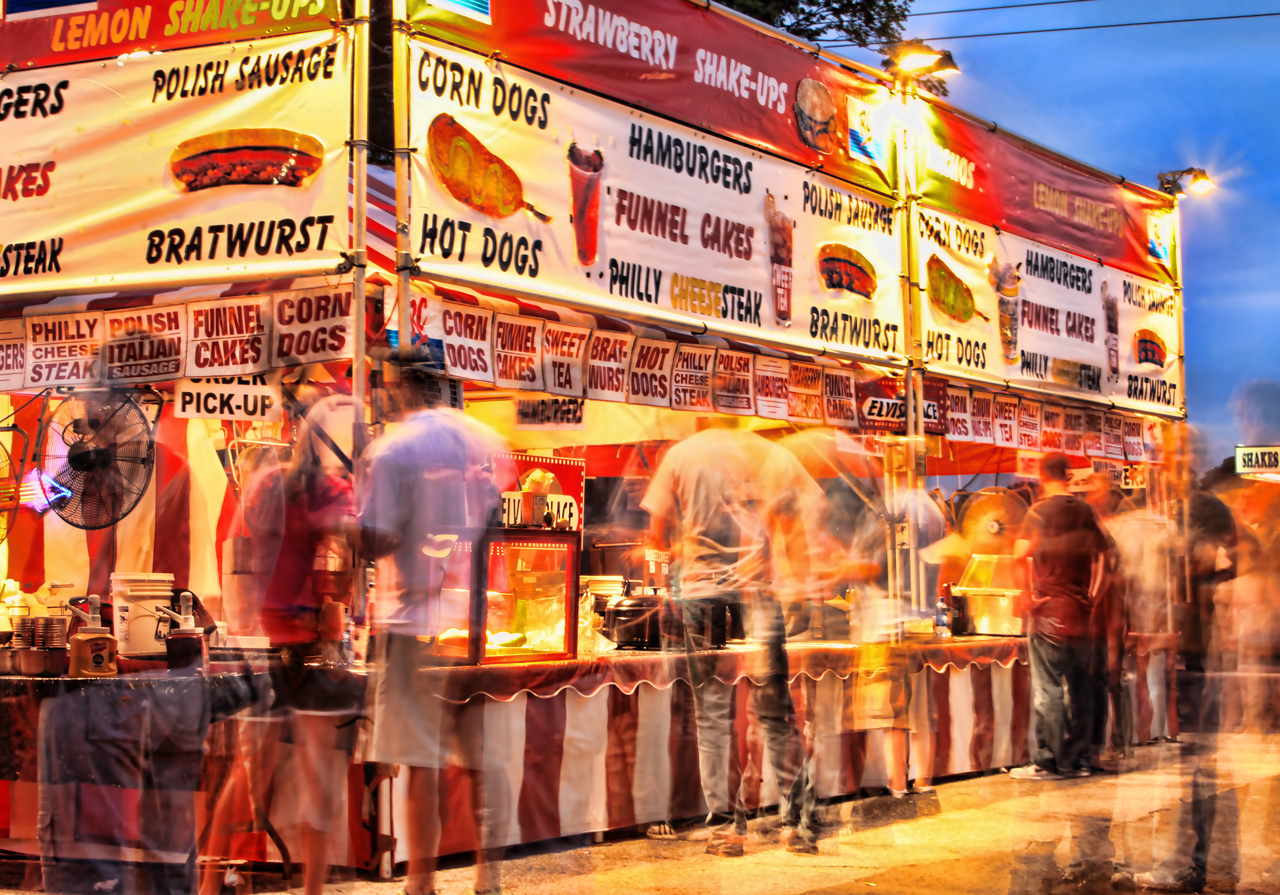This captivating time-lapse image captures the bustling scene at a vibrant food booth at a fair or carnival. The red banner at the top prominently advertises "Lemon Shake Ups" and "Strawberry Shake Ups," while a white banner just below it details an array of fairground delights including corn dogs, hot dogs, hamburgers, funnel cakes, Philly cheesesteak, bratwurst, and Polish sausage. Additional smaller signs reiterate offerings like funnel cakes, corn dogs, sweet tea, bratwurst, and hot dogs. Beneath these signs, an open counter enables workers to hand out food to the eager patrons on the other side. A red and white vertically striped table skirt at the bottom completes the festive look, reminiscent of classic carnival décor. The image uniquely features multi-exposure shots of people standing at the booth, giving them a ghostly, translucent appearance with a slight blur, conveying the continuous flow of customers throughout the day. The extensive signs and the array of cooking supplies behind the counter emphasize the busy and lively nature of this popular food destination.